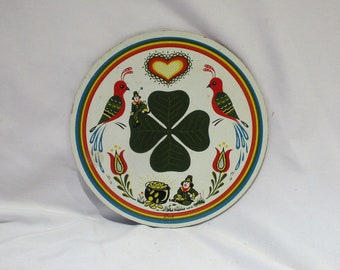This image features a round, white plate displayed on a white cloth backdrop. The centerpiece of the artwork is a black four-leaf clover, adorned with a small leprechaun figure perched on the left leaf. Above the clover, a heart with a yellow center, an orange middle layer, and a black outline stands prominently. Each side of the clover is flanked by a vibrant red bird, showcasing green and yellow patterned wings and a blue tail, all facing inward towards the clover. Below the clover, a scene unfolds with a second leprechaun sitting adjacent to a black pot of gold. Further decorating the lower section of the plate are two red tulips, each with lush green leaves. The entire composition is encircled by a red and green border, enhancing the intricate details against the clean white background of both the plate and the cloth.